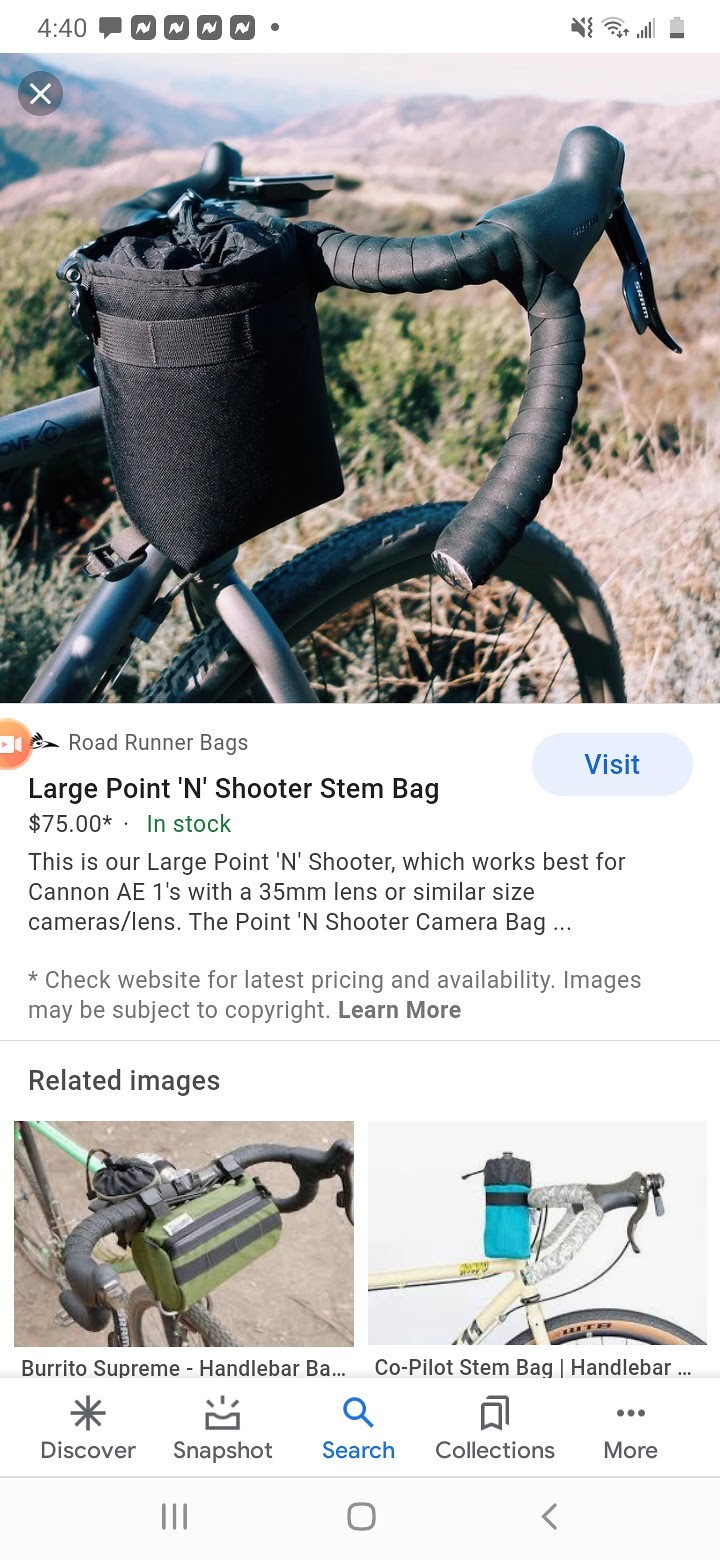This vertical rectangular image, likely a screenshot taken from a cell phone, depicts a product listing in a Google image search. At the top of the screen, indicators for time (4:40), text, notifications, silent mode, Wi-Fi, and battery status are visible. The main image features the front of a bicycle with black handlebars and a black bag attached to the handlebars. The bicycle is set against a mountainous background with a mix of dark green foliage and brown, white, and gray seasonal foliage.

The on-screen text highlights a product from Roadrunner Bags, specifically the "Large Point and Shooter Stem Bag" priced at $75 and noted to be in stock. This bag is described as being well-suited for Canon AE1s with a 35mm lens or similar-sized cameras. Additional text advises checking their website for the latest pricing and availability, noting that the images may be subject to copyright.

Below the main image, there are related images featuring close-ups of bikes with different handlebar bags: an olive green pouch with black and gray stripes and a cyan pouch with a black lid and stripe. The navigation options include "Discover," "Snapshot," "Search," "Collections," and more, along with various icons such as a star, a rectangle with lines, an hourglass, and ellipses. A directional arrow pointing to the left is also present at the bottom right corner.